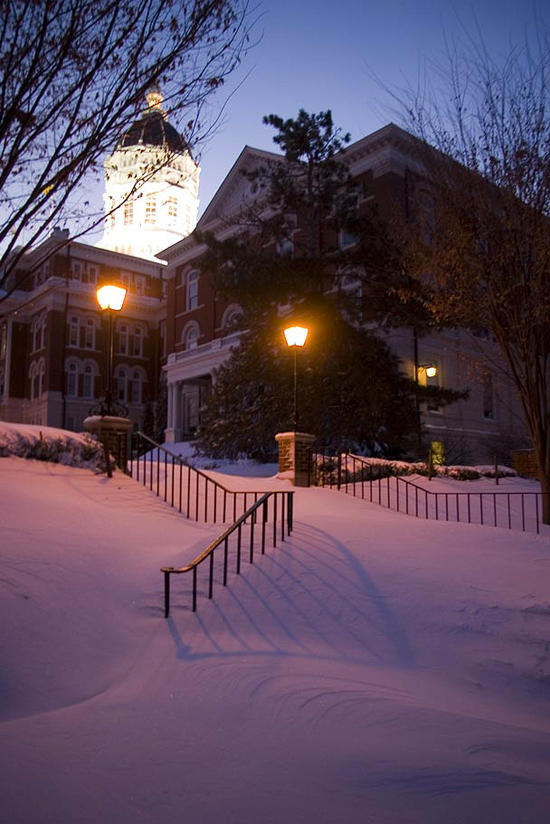This vertical photograph captures an impressive, large building complex in a snowy suburb during early evening. The ground is blanketed with snow, obscuring an L-shaped staircase with wrought iron handrails that ascend to the buildings. The main structure, a tall brick-faced edifice with white trim around its arched windows, stands three or four stories high and features multiple rows of double windows. A distinctive domed tower rises from the building's roof. To the right side of the shot, another structure is partially visible, sharing similar architectural features, including a bright white steeple that glows against the darkening sky. Illuminated street lamps on towering black poles sit atop sturdy brick pillars, casting a warm glow on the snow-covered surroundings. Additional details include leafless trees and a large fir tree near the second building, alongside a prominent bush laden with snow. The entire scene exudes a tranquil winter atmosphere, with the majestic buildings possibly serving as schools, churches, or significant residential properties.